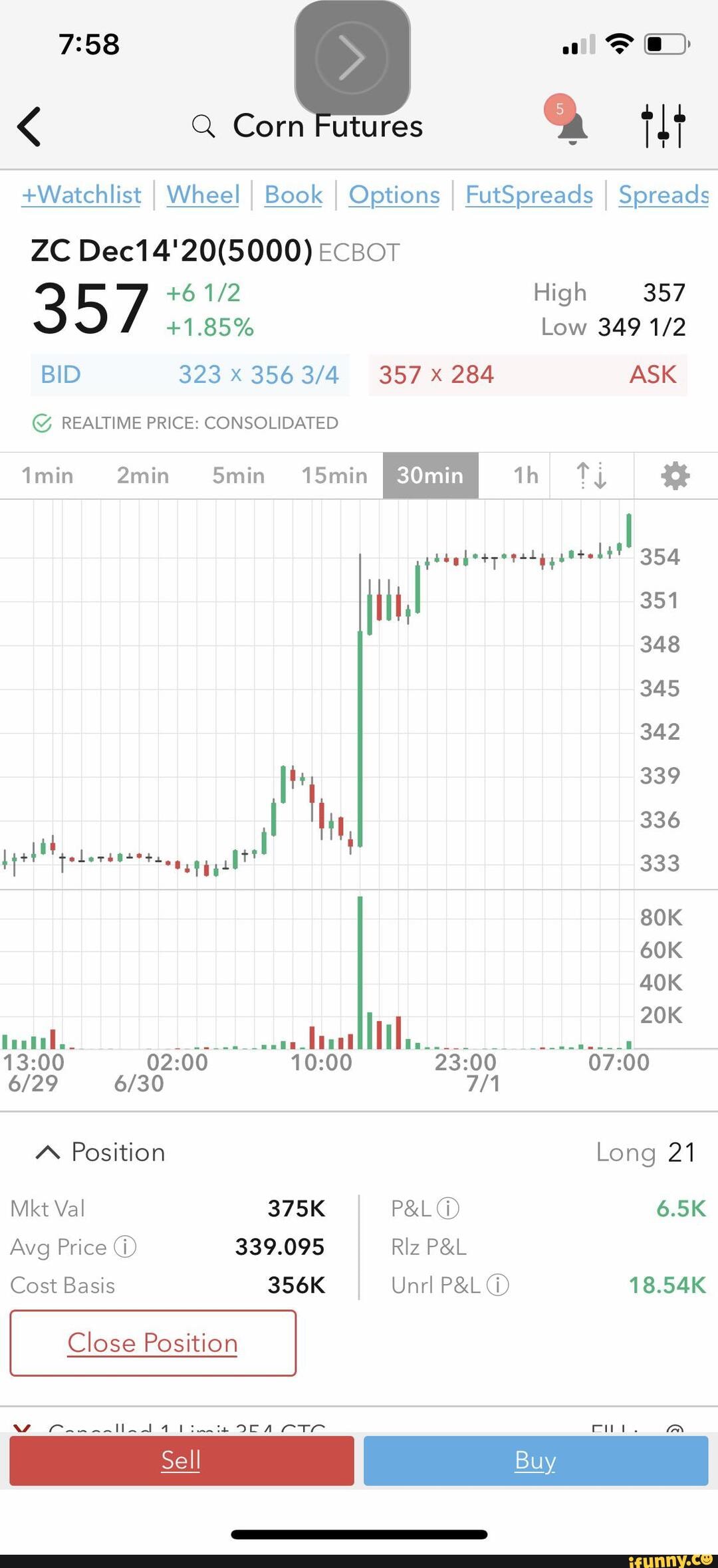This screenshot of Korn Futures prominently features a variety of details. At the top left corner, the number 758 is displayed. Adjacent to this, on the right, are icons indicating signal strength, Wi-Fi status, and battery level. Dominating the center of the screen is a right-arrow icon within a rounded rectangular box. Directly below this, the text "Korn Futures" is visible, accompanied by a bell icon with a red circle containing the number five, indicating notifications.

Further down, several sections appear in blue underlined text, including "Watchlist," "Wheel," "Book," "Options," "Foot Spreads," and "Spreads." Beneath these sections is the label "ZC December 14, 2020 (5000 ECBOT)," specifying the contract details. 

The main part of the screen is occupied by a graph presenting fluctuating red and green lines, which likely represent market trends or price changes over time. At the very bottom, there are two distinct buttons: a red "Sell" button on the left and a blue "Buy" button on the right, offering quick trading options.